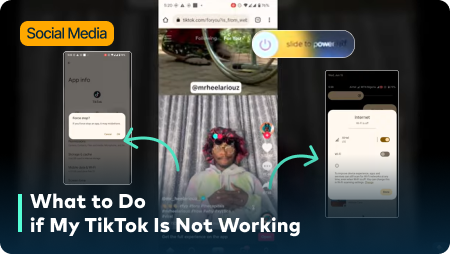The image depicts a detailed tutorial on troubleshooting TikTok issues, presented in a screenshot from a smartphone. At the center of the image is a TikTok video featuring a content creator, possibly an African American woman with curly hair, explaining, "What to do if my TikTok is not working." Surrounding this central screenshot are smaller, less legible images illustrating various troubleshooting steps. These steps include going into the smartphone settings, adjusting Wi-Fi settings, toggling the connection on and off, and restarting the phone. The presentation is somewhat playful, aiming to simplify the troubleshooting process for TikTok users experiencing connectivity or performance issues.